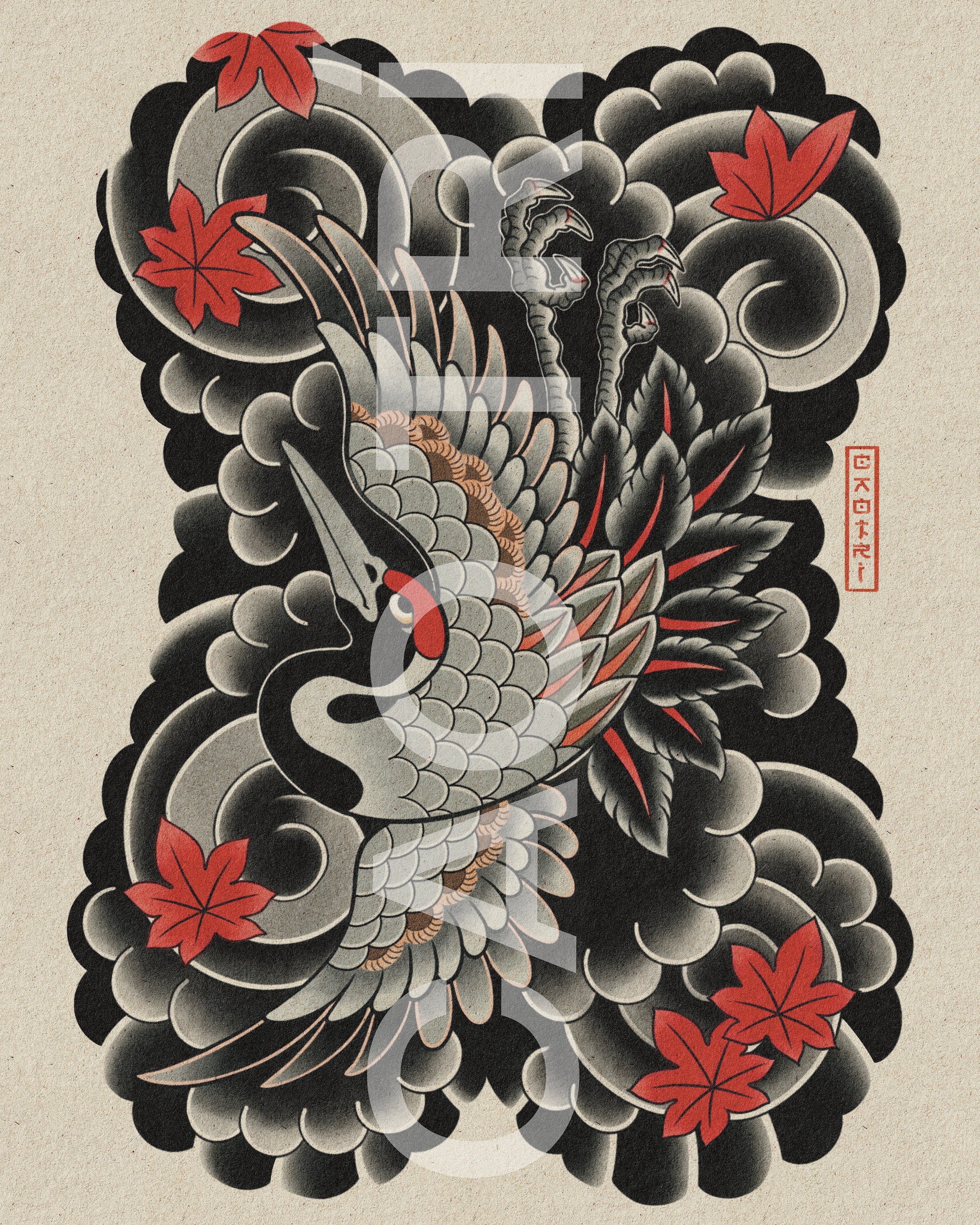The artwork presents a visually intricate composition featuring a centrally positioned bird, possibly a crane, drawn in an Asian style, likely Japanese or Chinese. The bird exhibits black feathers with red stripes and appears to have its wings spread, showcasing detailed outlines of each feather. The background is a tan, mottled canvas adorned with swirling shapes and sparse, red maple leaves dispersed across the scene. The image uses a limited palette of black, red, gray, and white, with some subtle tan accents in the bird's feathers. Additionally, there is vertical Asian text, possibly Chinese, on the far right side of the image. Amidst the dynamic patterns and elements, faded gray words are seen, which could signify a brand or artist's name, adding layers of mystery and intrigue to the already busy and enigmatic artwork.